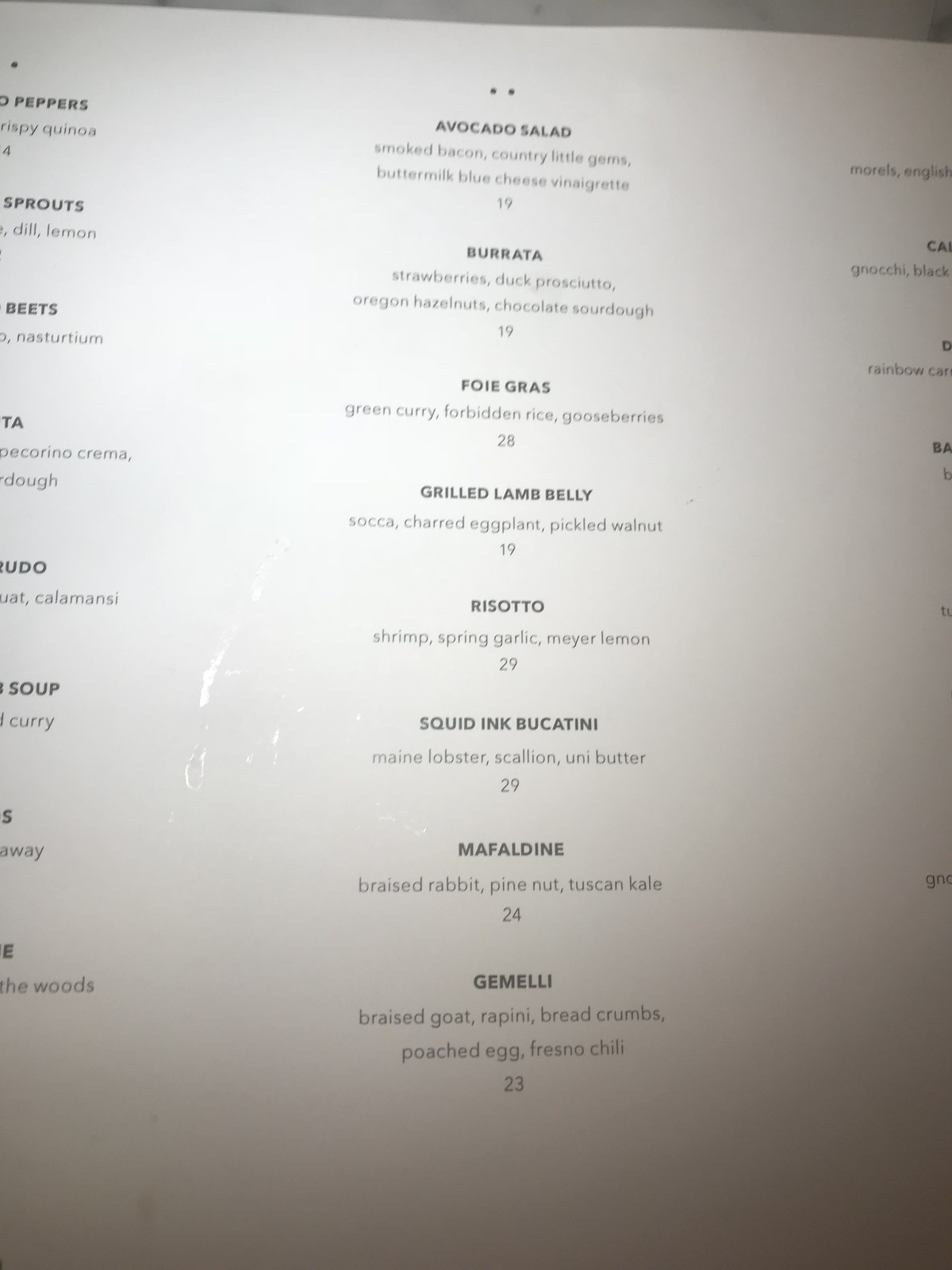This photo captures a partial view of a restaurant menu that has been shot in portrait orientation while the menu itself is laid out in landscape orientation, resulting in many of the items being cut off. The menu is divided into three columns, but due to the angle of the photo, only one full column in the center is clearly visible, with limited visibility of the columns on the left and right. 

In the center column, which is displayed against a white paper backdrop with subtle shadowing at the bottom, the items are listed in bold black font. The center column includes the following dishes: 

- Avocado Salad with ingredients listed, priced at $19
- Burrata with ingredients listed, priced at $19
- Foie Gras with ingredients listed, priced at $28
- Grilled Lamb Belly, priced at $19
- Risotto with ingredients listed, priced at $29
- Squid Ink Buccatini with ingredients listed, priced at $29
- Mafaldine, priced at $24
- Gemelli, priced at $23

The left column is partially visible, with only fragments of words like "peppers," "sprouts," "beets," and "soup" discernible. The right column is even less clear, with barely visible parts of food descriptions and a few words such as "milky," "black," and "rainbow." Overall, the photograph’s composition makes it difficult to get a complete view of the menu offerings.